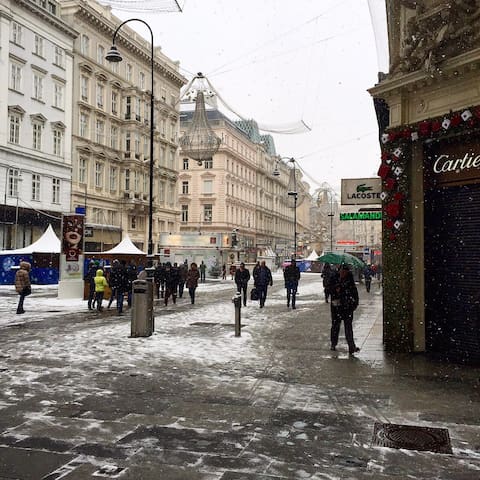The image depicts a bustling city street scene, likely in a European town, characterized by classical architecture and large six-story buildings flanking both sides of the street. It appears to be winter, as there is a dusting of snow on the ground and partially melted snow between the paving stones. The street is lively with numerous people dressed in coats, walking and carrying umbrellas.

Adding to the festive atmosphere, Christmas lights are elegantly strung between buildings, with chandelier-shaped lights hanging down the length of the street. Small kiosks and tented stalls line the pathways, suggesting a street fair is in progress. Prominent shops such as Cartier, Lacoste, and Salamander are visible, with their signs prominently displayed above doorways.

Additional details include a garbage can situated along the street and a banner or poster with possible musical instrument imagery, contributing to the vibrancy of the scene. The crowd’s presence and the various decorative elements emphasize the lively and festive nature of this cityscape.